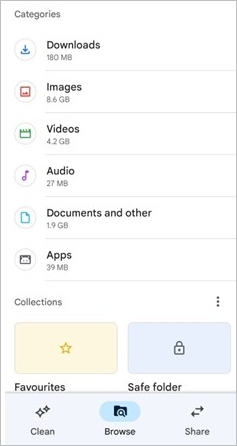This image is a screenshot of a search interface, organized by categories and collections. At the top, the word "Categories" is shown in gray text. Below it, listed in both black and gray text, are the different types of files along with their sizes: "Downloads, 180 MB," "Images, 8.6 GB," "Videos, 4.2 GB," "Audio, 27 MB," "Documents and others, 1.9 GB," and "Apps, 39 GB." Each category is accompanied by a distinct icon, such as a purple musical note for audio files and a blue file folder for documents and others.

Beneath the categories, there are two rectangular boxes: the one on the left is light yellow, and the one on the right is light blue. Above these boxes, the word "Collections" is displayed. The light yellow box features a yellow star icon in its center, labeled "Favorites," while the light blue box, labeled "Safe folder," contains an unspecified icon. 

Below these boxes, a menu presents three options — "Clean," "Browse," and "Share" — each with corresponding icons positioned above them.